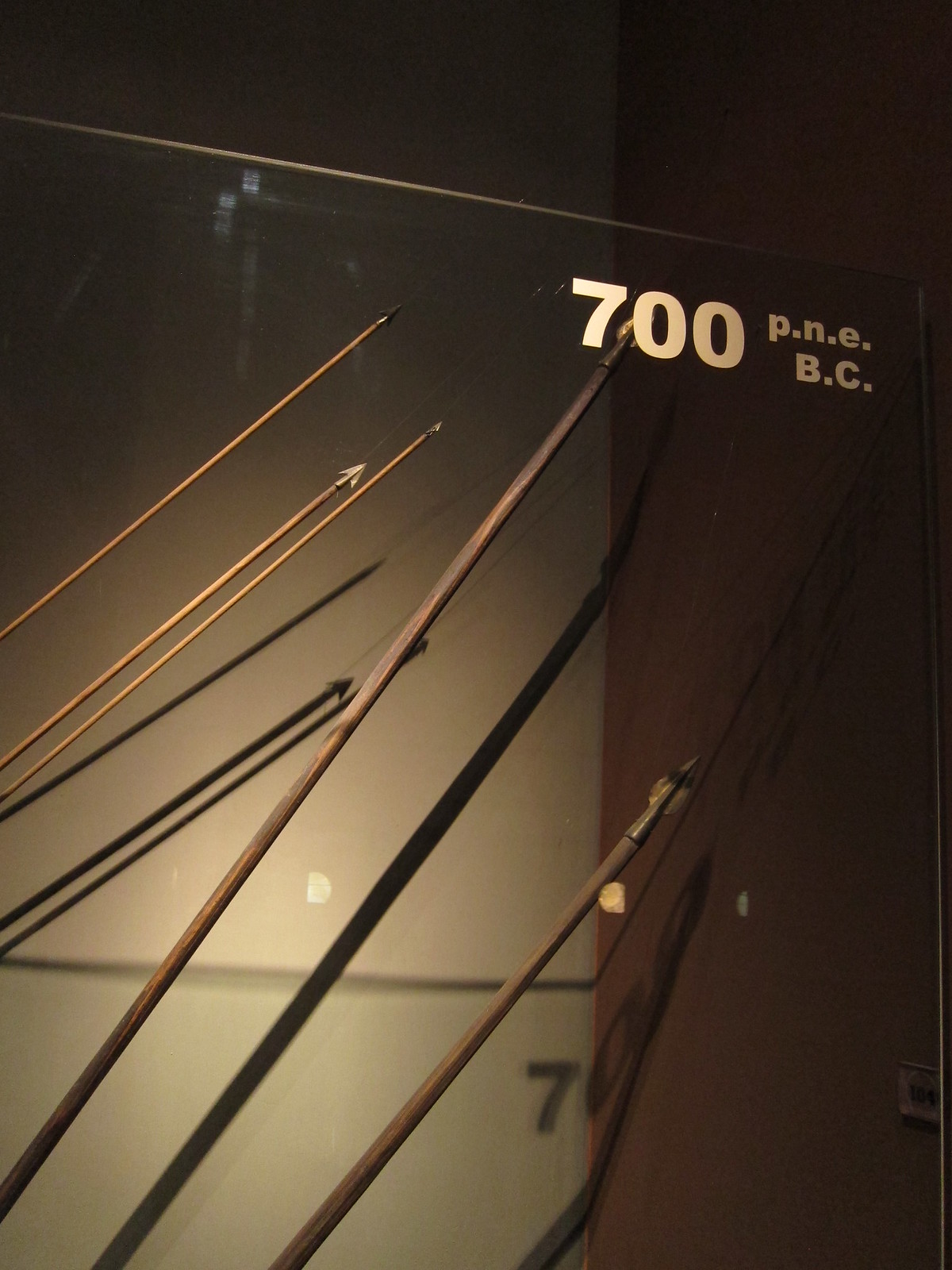This detailed color photograph, likely taken inside a museum under dark sepia-toned lighting, captures an array of spear or arrow tips displayed in a glass case. The tips, ranging from thin and small to long and thick, are crafted from wood and feature sharp silver points. These arrows are oriented from the bottom left to the top right of the image. At the top right corner of the glass display case, white lettering spells out "700 P.N.E" with "B.N.C" beneath it. Reflections on the glass from the lighting create a mid-line shadow featuring the number "7" and mirror the surrounding objects, enhancing the depth and historical ambiance of the display.